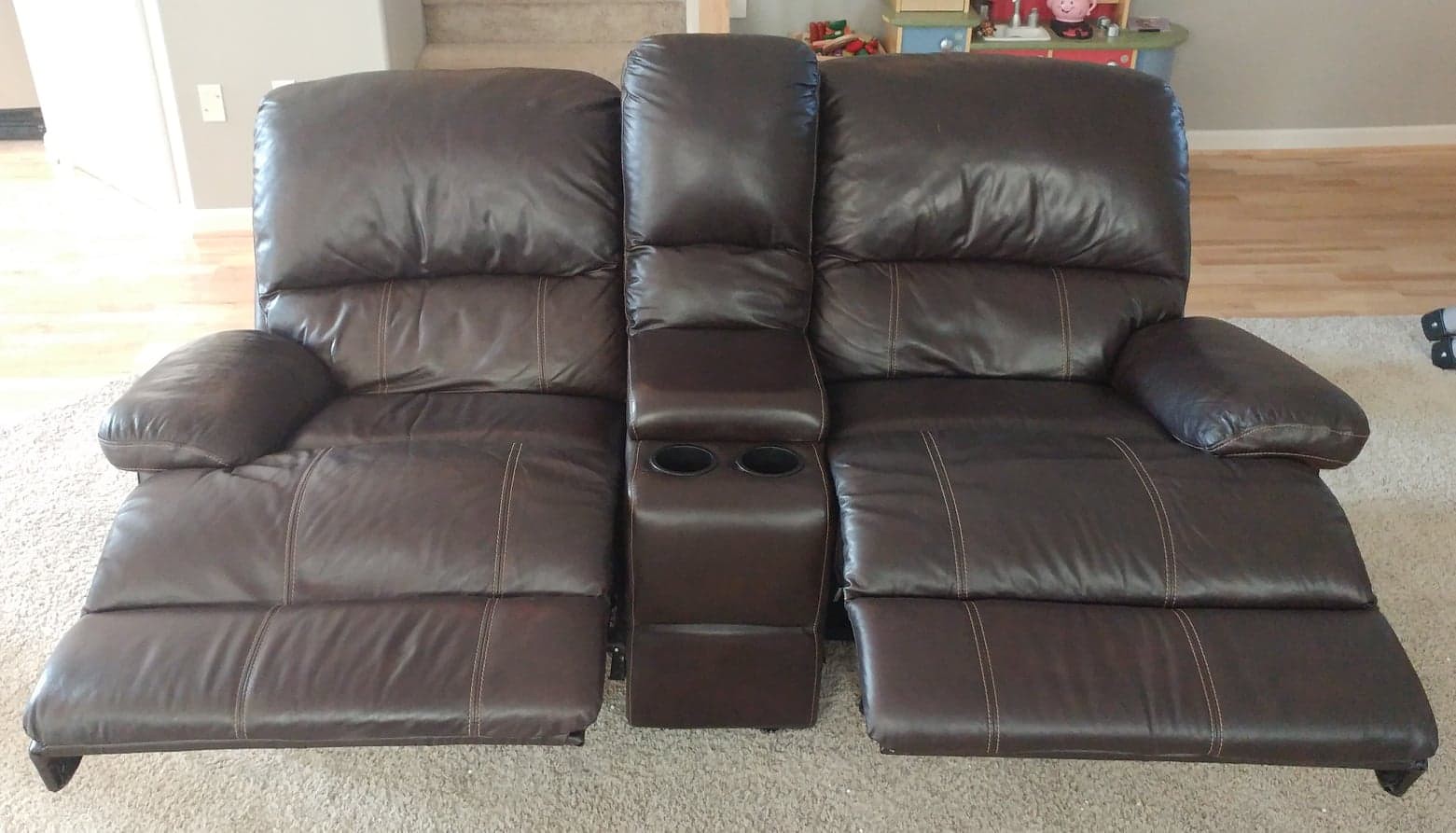This is a photograph of a cozy man cave featuring a dark brown leather reclining loveseat with contrasting lighter brown stitching, flanked by two matching Lazy Boy brown leather recliners. The loveseat, equipped with extended leg rests and plush armrests on either side, also boasts a central console with two black cup holders and a flat surface for placing items. These seating arrangements rest on a light gray carpet, which transitions into a light brown wooden floor. Behind the seating area, there's a gray wall with white crown molding and tan carpeted stairs ascending directly. To the right of the chairs, a colorful children's toy cabinet in reds and blues adds a playful touch. The photo, taken from an elevated angle, also captures a bright light in the top left corner, suggesting illumination from a window or nearby room. A hint of a black shoe peeks into the frame, adding a subtle human element to the scene.